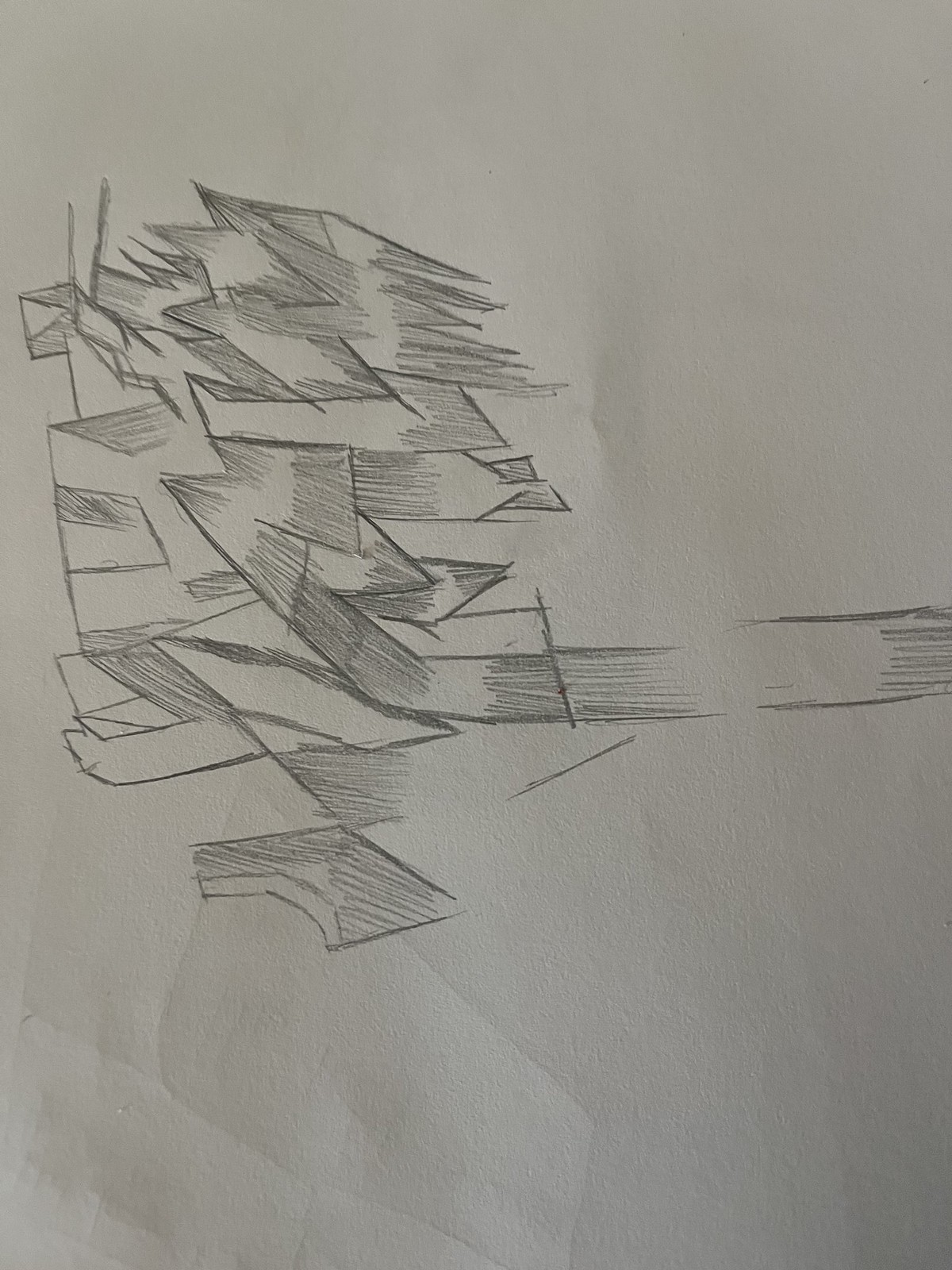This photograph captures an abstract pencil drawing on a slightly wrinkled white paper. The artwork features an intricate arrangement of geometric shapes, primarily squares and triangles, densely clustered on the left side. Some shapes deviate from typical forms, creating an intriguing mix of oddly-made figures. Each shape is meticulously shaded with horizontal lines, adding a textured dimension to the piece. The composition extends dynamically toward the right, creating the illusion of movement. Notably, indents from another drawing process are subtly visible on the paper, hinting at previous uses. Amidst these shapes, faintly resembling a creature with possible antennae and a tail, the drawing evokes a sense of organic, yet structured chaos.